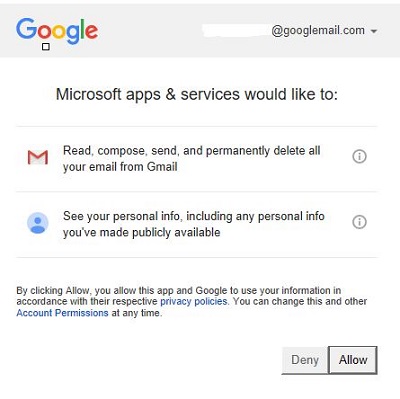A low-quality screenshot depicts a typical interface used for connecting an app with Google, specifically Gmail. The interface features Google's multi-colored, sans-serif logo prominently displayed in the top left corner. In the upper right-hand corner, an email address is shown as "googleemail.com," which appears to be outdated compared to the more familiar "gmail.com." The personal identifier part of the email has been obscured for privacy.

The interface displays a title reading: "Microsoft apps and services would like to:" followed by a detailed request. The first request is represented by a Gmail icon and states that Microsoft apps and services would like to "read, compose, send, and permanently delete all your email from Gmail." The second request is for permission to see the user’s personal information, including any publicly available info.

At the bottom of the interface, smaller text informs the user that by clicking "Allow," they are permitting the app and Google to use their information in accordance with their respective privacy policies. It also notes that account permissions can be changed at any time. Two buttons are provided for the user to respond: "Deny" and "Allow."